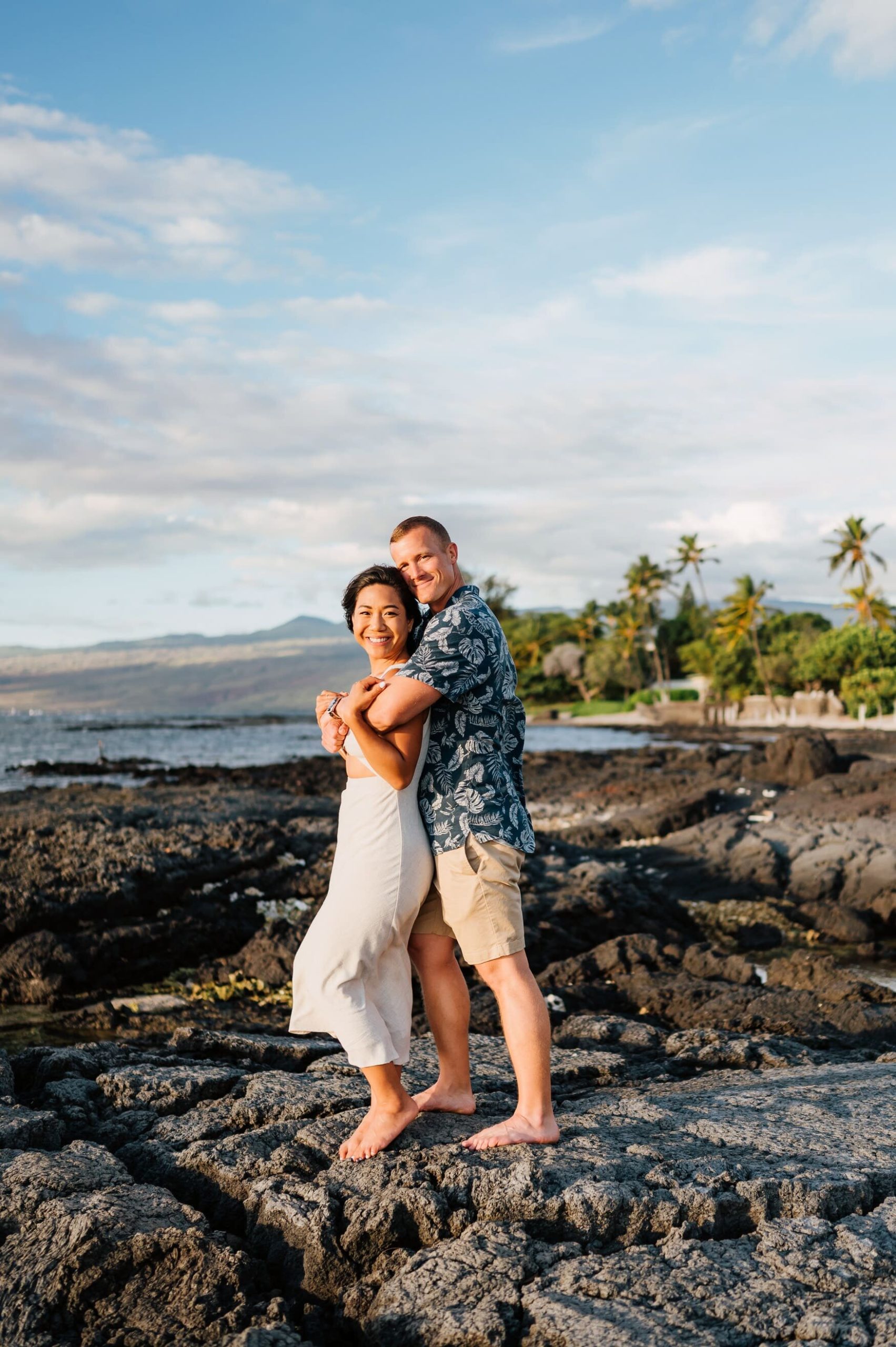This photograph captures a young couple standing on black volcanic rocks by a beach, likely in Hawaii. The woman, possibly of Asian or Pacific Islander descent, is on the left, wearing a long white dress that reaches close to her ankles. Her brown hair is pulled back. The man, a white male, is standing behind her with his arms wrapped lovingly around her waist. He is wearing tan khaki cargo shorts and a blue Hawaiian shirt adorned with white symbols. Both are barefoot, grounded on the rugged, hardened lava terrain.

The scene around them is lush and picturesque, epitomizing tropical paradise. To the right, there is verdant land with dense greenery and towering palm trees. Off in the distance to the left, hills rise subtly, hinting at volcanic origins. Hampered by a hazy sky, the background with possible volcanoes remains indistinct, blending into the soft blues overhead. Above them stretches a clear blue sky punctuated by a few scattered clouds, adding to the serene and romantic atmosphere of the photograph. The couple, both smiling warmly at the camera, appear joyful, possibly capturing a moment from their honeymoon or a special vacation.